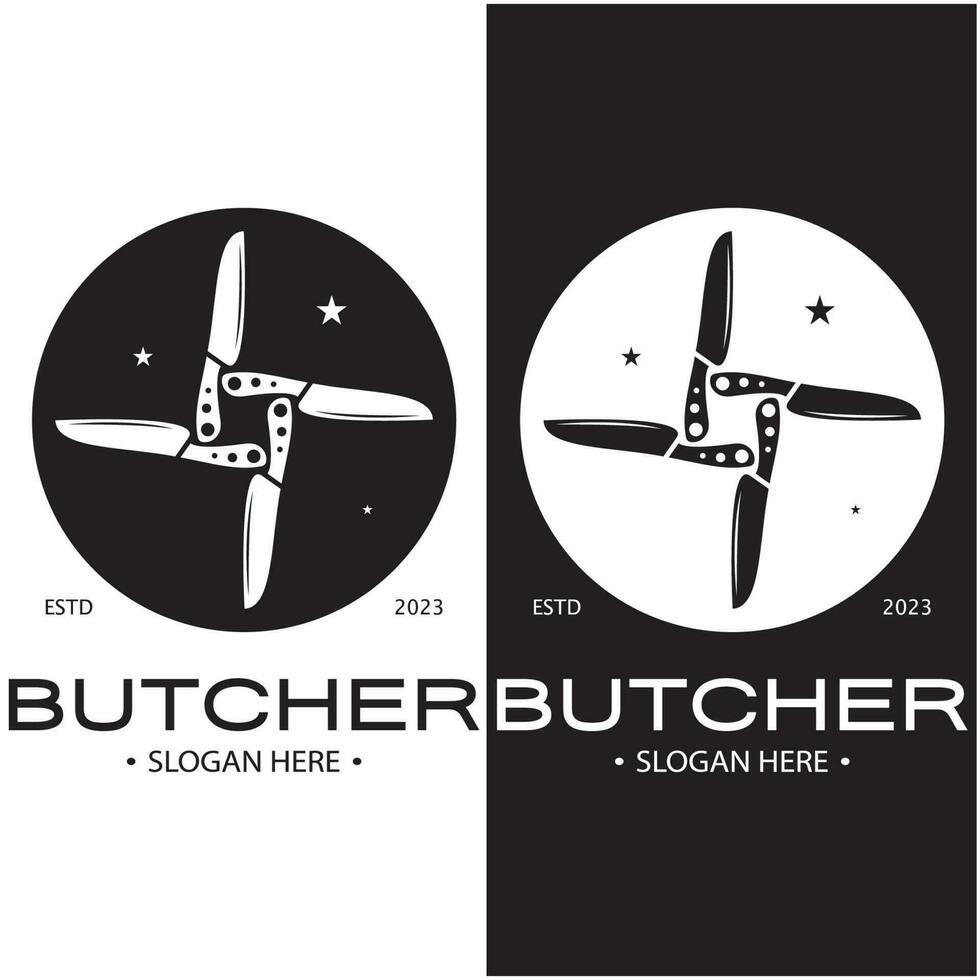This image features two side-by-side logos, presented in a black and white, inverse color scheme. The left logo has a white background with a central black circle, inside which are four white steak knives arranged in a star-like, square pattern, resembling a Chinese throwing star. Accompanying the knives are three small white stars. Below the circle, the text "ESTD 2023" appears, with "ESTD" on the left and "2023" on the right, all in black font. The prominent word "butcher" is displayed in black, with "slogan here" in smaller black font beneath it.

The right logo mirrors the left one but in an opposite color scheme, essentially a negative image. It has a black background with a white circle at the center. The four steak knives inside the circle are black, arranged in the same star-like pattern, with three black stars around them. Below the circle, the text "ESTD 2023" appears in white, with "butcher" and "slogan here" also in white text. The contrasting color schemes create a visually striking comparison between the two logos, emphasizing their similarity and subtle differences.